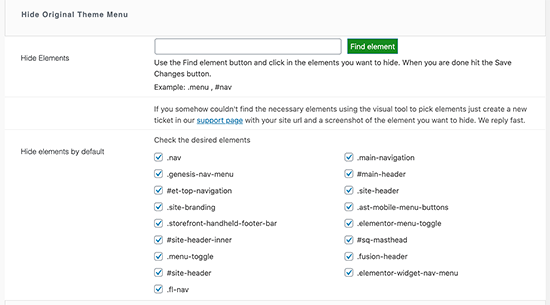This image, sourced from a website, prominently features a user interface related to element management themed settings. The interface is framed by a light bluish top border and light grayish side borders that fade to white as they descend. In the top-left corner, bold black text states "Hide Original Theme Menu."

The left side of the image contains a white background area where the text is displayed in black. It begins with "Hide Elements," followed by a two-inch gap, and then "Hide Elements by default" with no additional content beneath it.

To the right, a long rectangular box with a black border and white interior is positioned next to a green tab labeled "Find Element" in white text. Below this is a helpful instruction: "use the Find Element button and click on the elements you want to hide. When you are done, hit the Save Changes button."

Continuing down the page, an example menu is noted with the label "example menu, A to B." Immediately below it is a small instructional note in black: "if you somehow couldn't find the necessary elements using the visual tool to pick elements, just create a new ticket in our." The word "Support Page" follows in blue and is underlined, indicating a hyperlink. The instruction concludes with "your site URL and a screenshot of the element we want to hide. We reply fast."

Further down, another instruction in black reads "check the desired elements." Below this, there are nine squares— each containing a blue checkmark, representing various elements to hide. Similarly, on the adjacent right side, there are eight white squares, also featuring blue checkmarks and labeled with black letters inside them. This clean and methodically organized interface guide ensures users can effectively manage and hide web elements as desired.